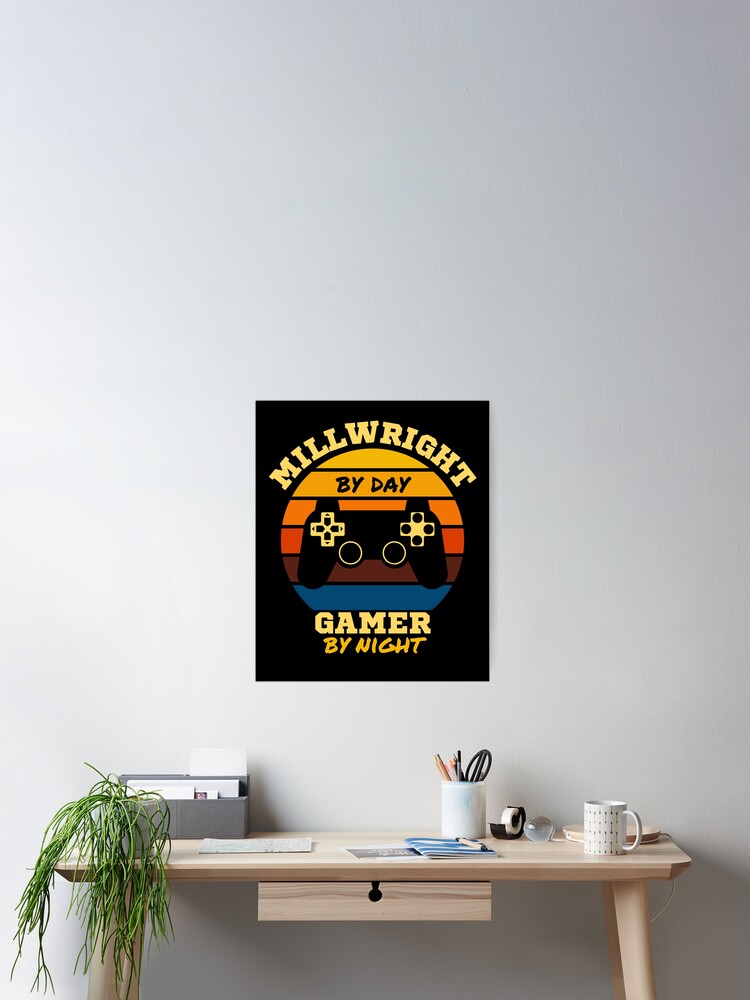This is a color photograph of a very modern, minimalistic wooden desk set against a white wall with a smooth gradient transitioning from light gray to darker gray. The desk is made of light wood and features a small slide-out drawer underneath. On the left side of the desk, there is a small green plant with leaves hanging over the edge. In addition, the desk holds a white, adjustable, and minimalistic lamp, a tape dispenser, a coffee cup, and another white cup without a handle containing various utensils like pencils and scissors. Papers are scattered on the desk, and there's a gray organizer box designed for holding mail or other office necessities. Above the desk on the wall hangs a black poster with the text, "Millwright by day, Gamer by night," accompanied by a colorful mosaic sun behind a gaming controller. The desk is neatly organized, reflecting a clean and modern aesthetic.